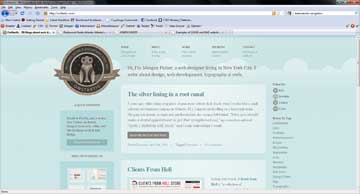This screenshot is highly compressed, rendering the text nearly illegible. The visual layout features a top border in black. In the top-right corner, a red square is followed by a grey square. On the left side, about two inches in from the edge, there is a grey strip.

The image shows numerous black-lettered texts, none of which are distinguishable. An inch-wide light grey band displays six indistinct black words, alongside several icons, and an extensive search bar spanning almost the entire width. 

Below this, there's a grey tab followed by a smaller search bar. Under these, six icons accompanied by unreadable black text are visible, with an additional row of seven icons beneath them. The interface includes several tabs: the first in white, and three subsequent ones in grey. Another search bar appears below these tabs.

Toward the lower section, the background shifts to light blue, evocative of a cartoon sky. Near the left edge, about an inch in, a grey crest featuring an owl is present. This crest has a banner with indecipherable letters around it.

To the right of the crest, there are five sets of illegible black text, each with accompanying information lines. A bolded black paragraph is followed by a grey tab with white letters. Under the owl crest, a light blue square with illegible text is seen alongside a light blue tab. Another light blue square, containing white squares, sits beneath it. The content within these elements remains unclear.